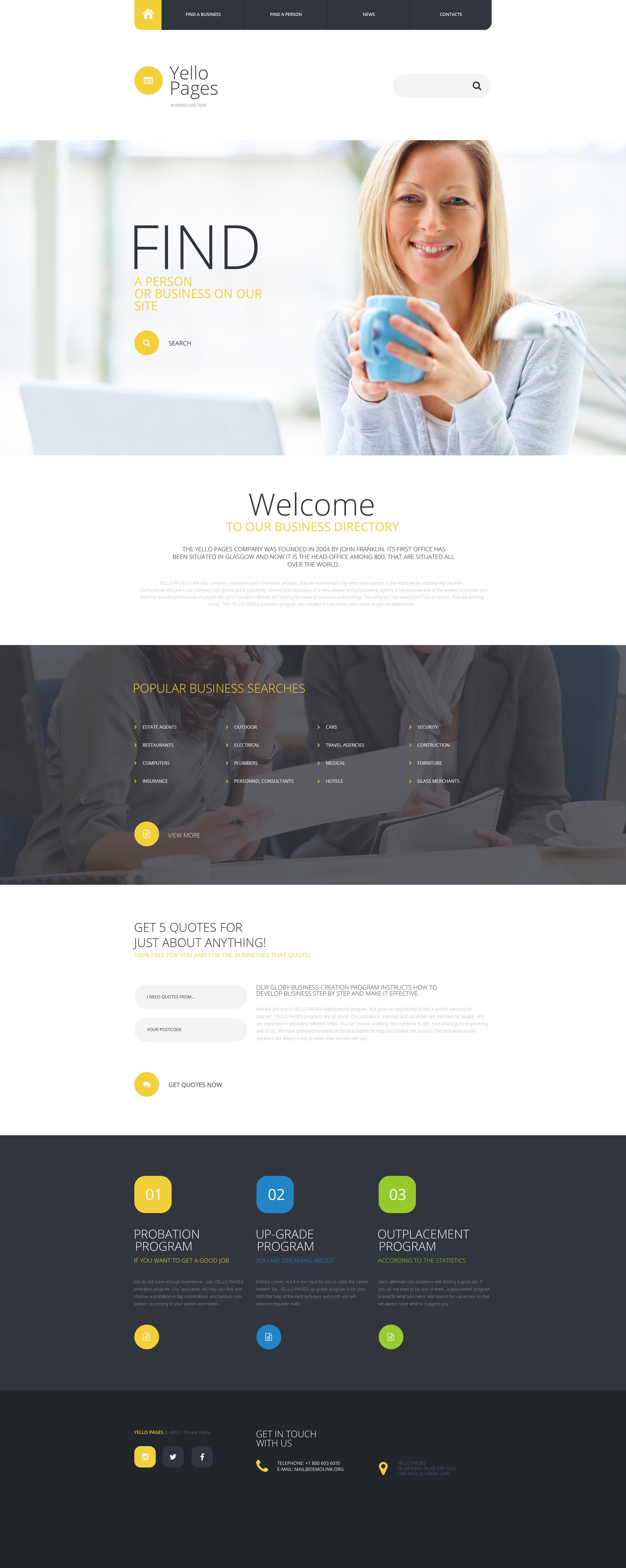This image captures a screen from the Yellow Pages section. At the top, there's a yellow emblem featuring a white page-like icon. To the right of this emblem, the words "Yellow Pages" are displayed in bold black text. Below this heading, an image of a woman holding a blue coffee cup with both hands near her head is prominently featured. She is smiling and sitting in front of a computer and a desk lamp.

The text on the screen includes the phrase "FIND" in large, capitalized letters, followed by "a person or business on our site" in a slightly smaller font. Adjacent to this text is a white magnifying glass icon set inside a yellow circle, symbolizing the search function.

Further down, the screen reads, "Welcome to our business directory," and provides a brief history of the Yellow Pages company, mentioning that it was founded in 2004 by John Franklin. The text continues, indicating that the first office was located in Glasgow, and it is now the head office among 800 offices worldwide.

As the viewer continues to scroll, the screen highlights "Popular Business Searches" and promotes the feature of getting five quotes for a wide range of services. The information extends further down, offering more details and navigation options.